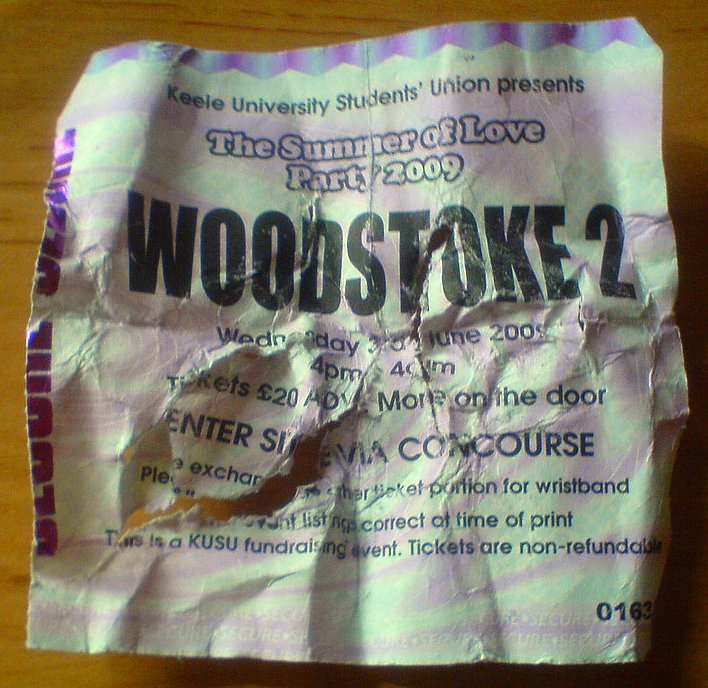This detailed photograph showcases a torn and tattered concert ticket stub laid on a wooden table. The table is brown and wooden, and though visible in the background, all attention is drawn toward the crumpled, square-shaped ticket in the foreground. This ticket, seemingly retrieved from someone's pocket, is adorned in a unique blend of white and swirling purple colors with bold black text. The ticket reads, "Keele University Students Union Presents the Summer of Love Party 2009 Woodstock II." Additional text indicates the event took place on a Wednesday, June 3rd, 2009, from 4 p.m. to 4 a.m., and the ticket cost 20 pounds. The creased and torn paper includes other entry details, but they are less legible due to significant wear, including a large tear through its center.